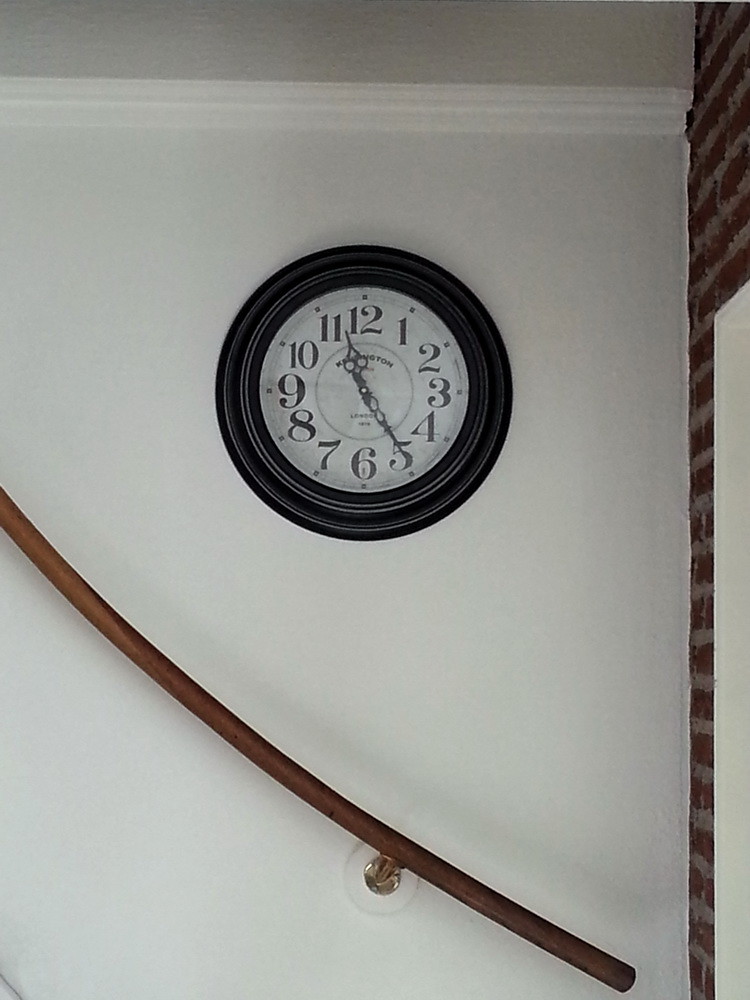A striking image captures a classic wall clock with a black frame and white face, prominently displaying black numbers and minute ticks. The clock hangs on a pristine white wall above a staircase, whose upward path is suggested by an angled wood railing secured by a gold-tone fixture. Although the stairs themselves are not visible, the direction of the railing, along with a parallel molding, hints at their ascent. To the right, a rustic brown brick wall with gray mortar provides a contrasting backdrop, enhancing the visual depth and charm of the scene.